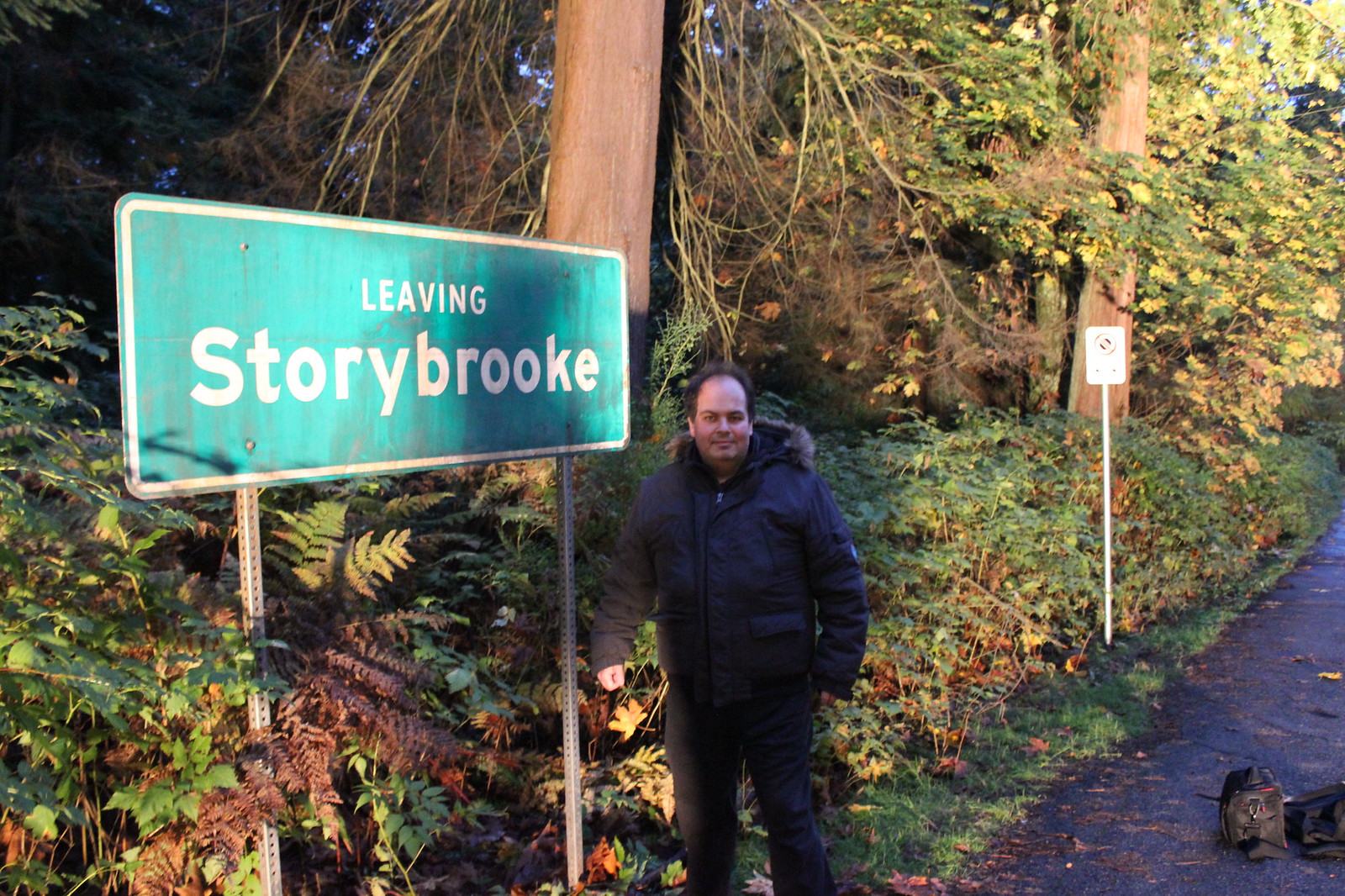In the detailed color photograph, a man is posing beside a green rectangular street sign that reads "Leaving Story Brook" in white text with a white border. This sign is mounted on two silver perforated square poles. The man, dressed in black pants and a black parka with tan-colored fur trim around the hood, stands in the center of the image. He has the hood down and is staring directly into the camera with a smile on his face. To his right, a wet, glistening gray asphalt road is scattered with various dead leaves, while a black duffel bag and possibly a black backpack are visible on the ground near him. On the left side of the photograph, the road's edge transitions into short green grass, leading to a forest area dense with tall green ferns and numerous trees with abundant leaves and branches. The bright sunlight highlights both the man and the foliage, casting a sunny, vibrant atmosphere over the entire scene. A smaller, slightly blurry warning sign is also present behind him amidst the greenery. The overall setting conveys a countryside ambiance with lush natural surroundings.